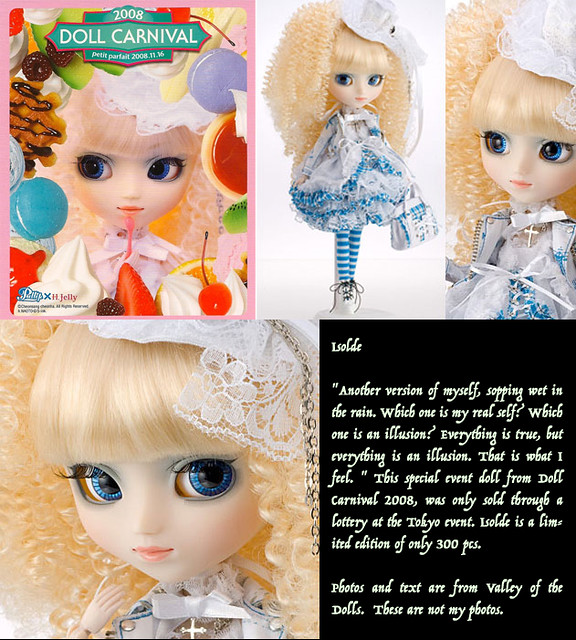The image is a composite layout showcasing a special event doll from the Doll Carnival 2008. At the upper left, a magazine cover features a doll adorned in a white veil and a white dress, accompanied by illustrations of cherries, strawberries, and raspberries. Centered at the top is the title "Doll Carnival 2008." Next to this, the middle section features three rectangular photos of the same doll from various angles. The doll, reminiscent of a Bratz doll but unique in its own right, dons a lacy white dress with blue trim that poofs out in a fit-and-flare style, descending to her knees. She accessorizes with a matching lacy white and blue purse, blue striped tights, and white shoes with black laces. Her prominent features include large blue eyes enhanced with blue eyeliner and eyeshadow, high and fluffy crimped blonde hair, and a 1910s-style blue lacy hat. Below this, close-up images highlight her detailed facial features and the lace on her veil. On the bottom right of the image, white text reads: "I sold another version of myself, sopping wet in the rain. Which one is my real self? Which one is an illusion? Everything is true but everything is an illusion. That is what I feel." It is further explained that this special edition doll, named Isolde, was a limited run of only 300 pieces, sold exclusively through a lottery at the Tokyo event. The photos and text are courtesy of Valley of the Dolls, emphasizing that they are not the original poster's photos.